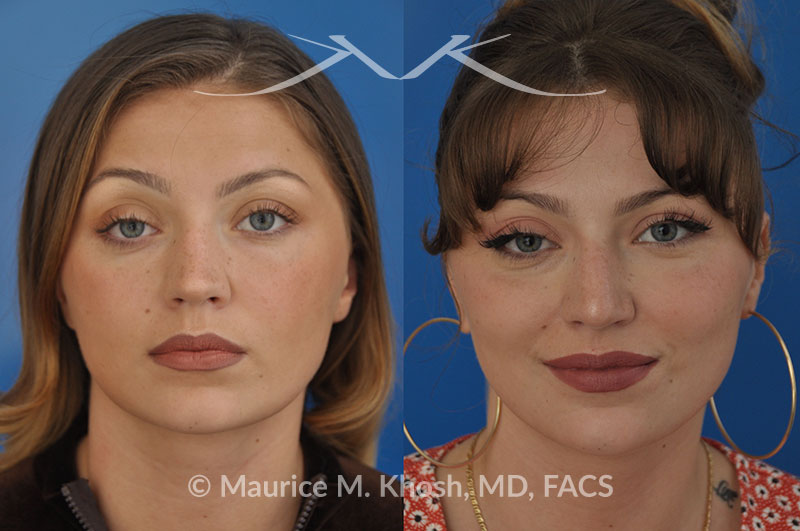This image features a realistic, side-by-side comparison of two females, likely the same person before and after a cosmetic procedure. The left image shows a woman with shorter brunette hair down, a black jacket with a gray zipper, pink lips, blue eyes (one slightly higher than the other), mismatched eyebrows, and freckles. She has a blank expression. The right image depicts the same woman with her brunette hair styled back in a bun, wearing big gold hoop earrings, a gold necklace, and a pink shirt. She is wearing heavier makeup, including pink lipstick and possibly false eyelashes, and is smiling slightly. Her eyes remain blue but are unnaturally separated. The top of the image features a silhouette with a backward and frontward facing letter "K," and at the bottom, the photographer's name "MAURICE M. KOCH, M.D., F.A.C.S." along with a copyright symbol is displayed in caps, indicating this may be related to a doctor's advertising for cosmetic enhancements.